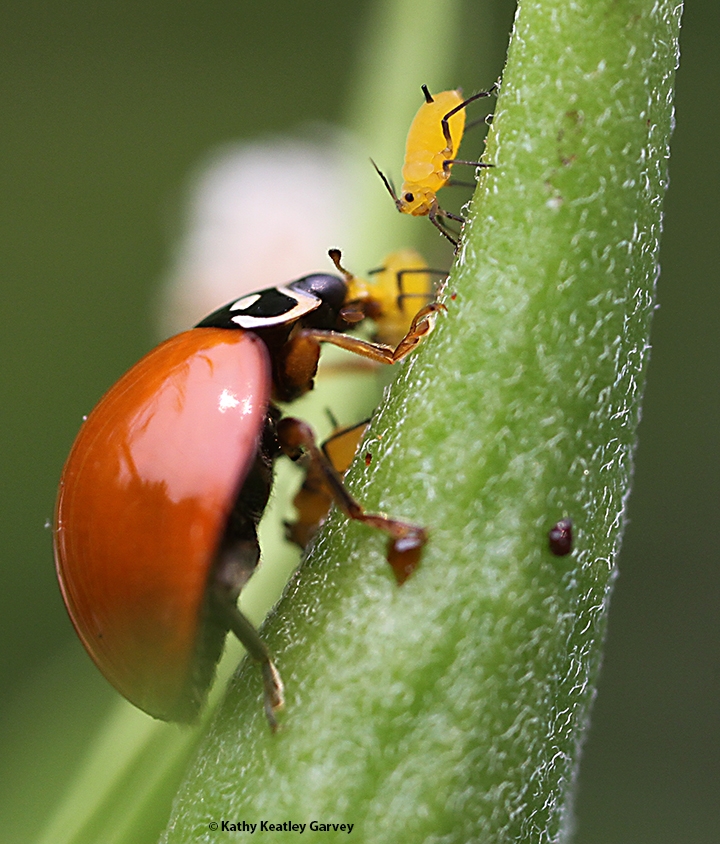This highly detailed macro photograph by Kathy Keatley Garvey features a red, spot-less ladybug with a shiny back, brown legs, and a black and white head, climbing up the green vertical stem of a plant. The close-up shot focuses on the ladybug's interaction with its environment, where it is seen facing and seemingly about to eat a smaller peachy-yellow aphid with black markings and two antennae. Additionally, the image includes two other blurred aphids in the background. The entire composition has a soft, blurred background that enhances the sharpness and detail of the insects on the plant. The copyright for Kathy Keatley Garvey is visible at the bottom of the photograph.